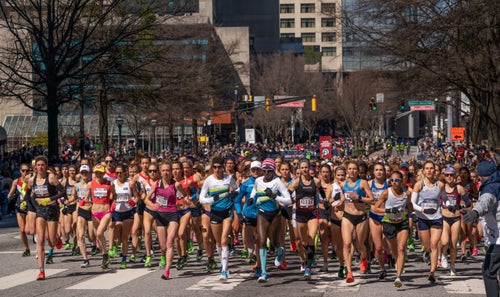A photograph captures the beginning of a marathon featuring a massive crowd of runners, predominantly women, who have just started their journey. The scene takes place on a wide city street devoid of visible signage identifying the event but is lined with large, brown buildings and an assortment of bare trees, indicating a winter setting. The participants, clad in athletic gear such as shorts, running shoes, and numbered bibs, flood the street, presenting a kaleidoscope of colors. Among these runners, a man stands to the right, arm outstretched, guiding the throng as they cross a white-striped crosswalk. Traffic lights punctuate the background, some shining green, while an orange road sign adds to the urban atmosphere. The energy and scale of this event, possibly the Boston Marathon, envelop the viewer in a dynamic and awe-inspiring display of human endurance and community spirit.